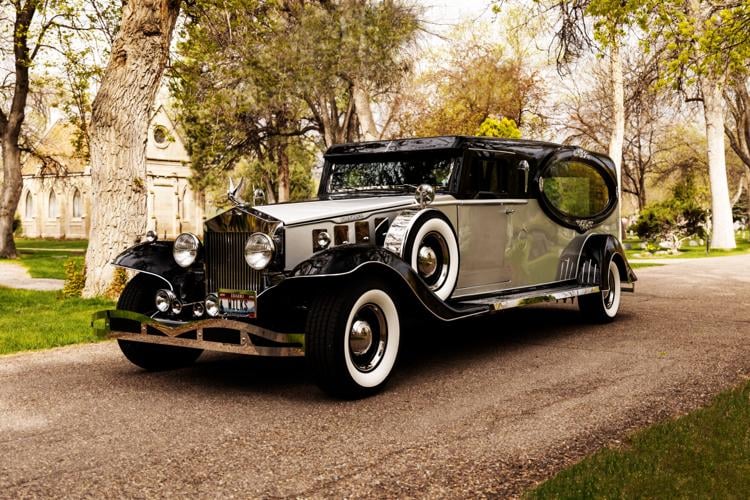The image depicts a vintage car, possibly from the 1920s or 1930s, parked on a gray and black road. The car, likely a Model T or similar type, is a light gray-tan color with a black top and black wheel wells. The car also features distinctive design elements such as a silver front bumper, a large chrome grill with round headlights, and a hood ornament that resembles an angel with wings. The tires have white outer walls with black centers and silver rims.

In the foreground, the road is bordered by green grass which extends diagonally upwards from the bottom right. The background features a white-grayish sky and a diverse array of trees, some green and others yellowish, standing on gray and brown branches. 

To the left of the car, there's a housing area with tan walls, white trim, and a tan or greenish rooftop. Additionally, a window with a black circular frame and a greenish hue can be seen at the rear of the vehicle. On the right-hand side of the image, there appear to be small graves and a possible mausoleum, suggesting the setting might be a cemetery. The license plate visible on the car reads "Wilkes" in black text against a white and blue background with a silver border.